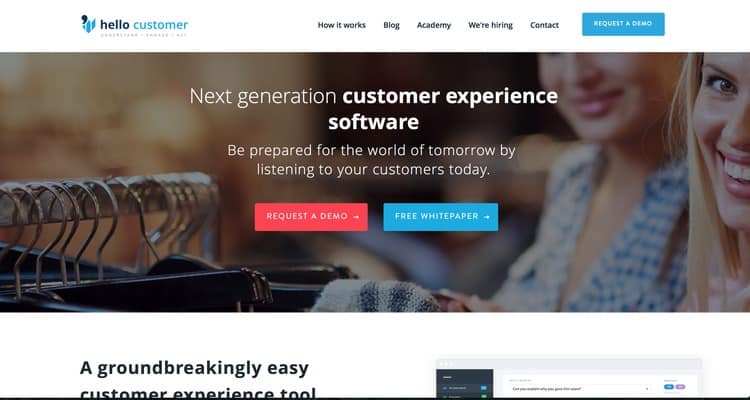Here is a cleaned-up and detailed descriptive caption for the image:

---

This image depicts the homepage of a customer experience platform, designed to enhance communication and service for users, reminiscent of a health insurance interface. 

At the top left, the brand name of the website appears alongside its emblem. "Hello customer" is presented in lowercase, with "hello" in blue and "customer" in light blue. The navigation menu on the right includes links labeled "How it works," "Blog," "Academy," "We're hiring," "Contact," all in black text, and a call-to-action button "Request demo" in a blue background with white text.

Below the navigation, the page transitions to a prominent image featuring two women. The woman on the right, with blonde hair, blue eyes, and a large smile, is slightly turned to the right. Beside her, another person, possibly a woman, is seen smiling subtly.

Centered on the image is a bold white text stating "next generation customer experience software," with "customer experience software" highlighted in bold. Below this, a tagline reads: "Be prepared for the world of tomorrow by listening to your customers today."

Underneath the tagline, there are two buttons: a red "Request a demo" button and a light blue "Free white paper" button, both in white text.

The image transitions into a white background showcasing a demo of the platform's interface. Towards the bottom of the page, partially obscured text reads: "A groundbreaking easy customer experience tool."

---

This complete and descriptive caption captures the key elements and the overall essence of the webpage as depicted in the image.